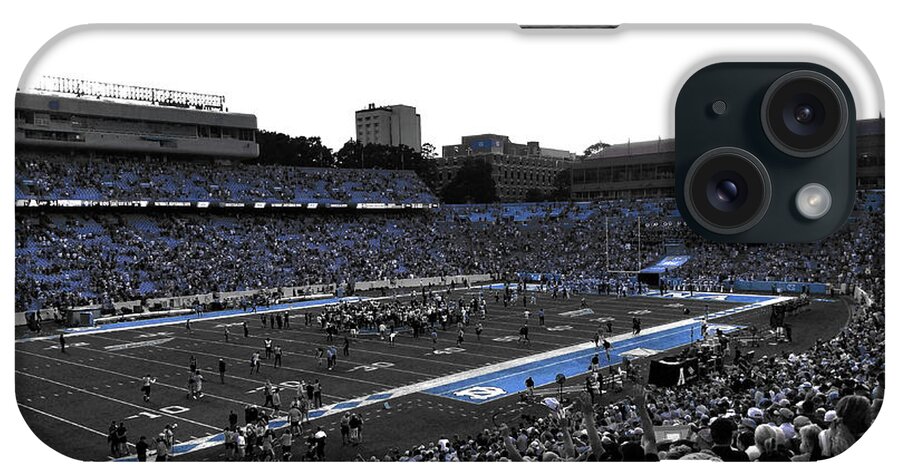This image depicts the back of an iPhone case featuring a detailed scene of a football game. The top half of the phone case, wider horizontally, includes a cutout for the camera in the upper right corner. The central image showcases a football field and stadium in a primarily black and white palette, accentuated with baby blue elements, including the stadium seats and a blue strip along the sidelines. This design element adds a pop of color against the backdrop of a white sky. The lower section of the case reveals a densely packed crowd, with one person notably raising both hands in the air, suggesting celebration or excitement, likely at the end of the game. Surrounding the stadium, you can discern various buildings in the distance, giving a sense of the larger environment beyond the field. This case captures the vibrant atmosphere of a football game, transforming it into a stylish and energetic accessory for an iPhone.